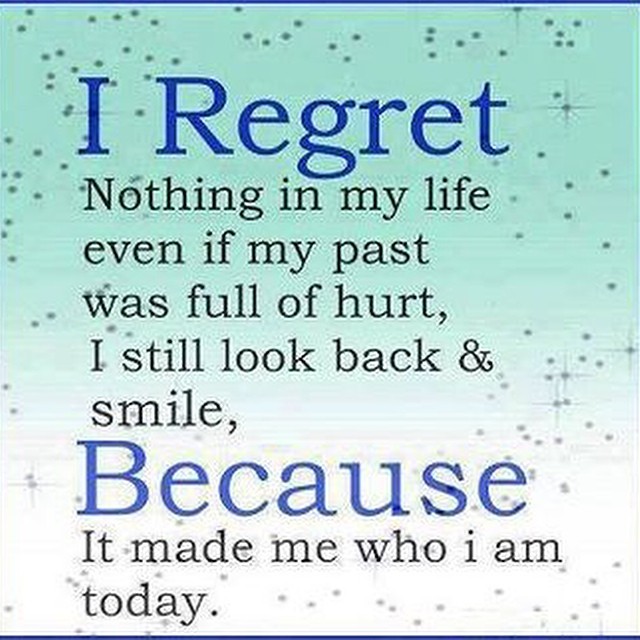The square image features a gradient background, transitioning from light blue or teal at the top to white at the bottom. The image is bordered by two horizontal blue lines, one at the top and one at the bottom. Scattered across the backdrop are small dot and star symbols, resembling sparkles or faded clipart, adding a subtle decorative element. At the center, the motivational quote is displayed, with the text "I REGRET" and "BECAUSE" prominently written in larger, blue font. The remaining text, "nothing in my life even if my past was full of hurt, I still look back and smile because it made me who I am today," is in smaller black font. This positive message emphasizes that despite past hardships, the individual holds no regrets as those experiences have shaped their current identity.